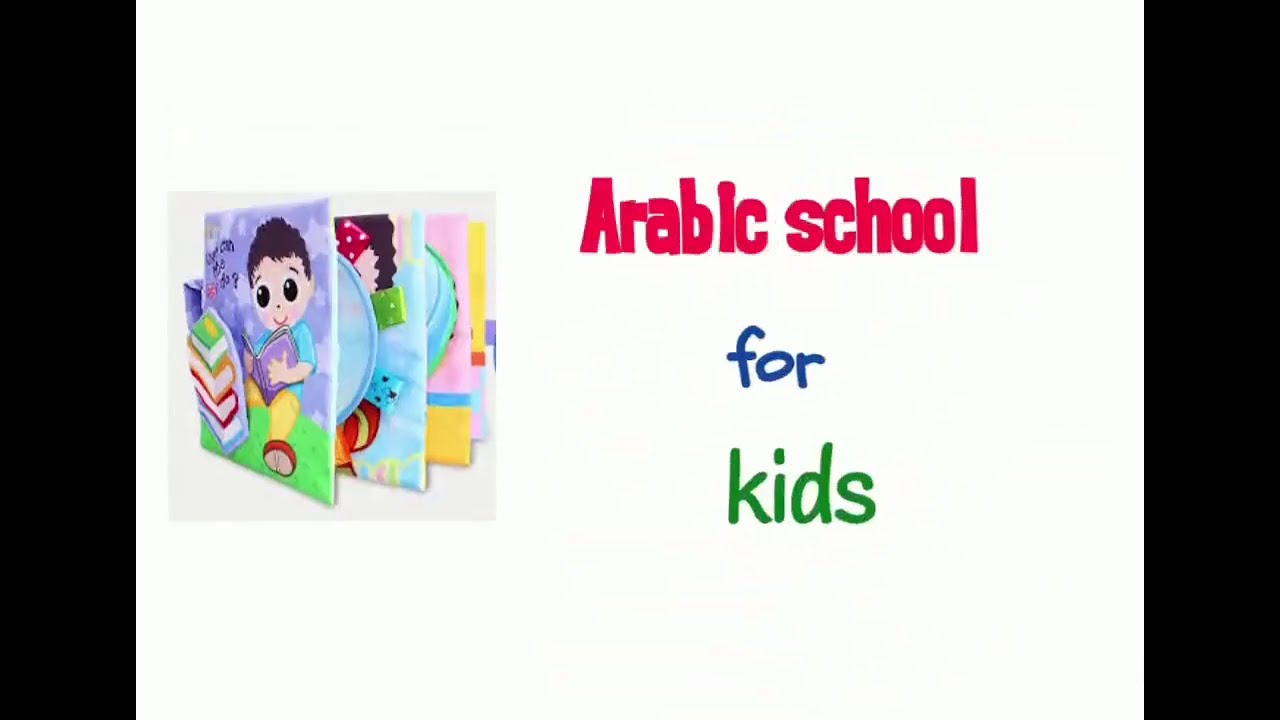The image features a promotional slide with a clear and vibrant text in the center, reading "Arabic school" in red letters, "for" in blue letters, and "kids" in green letters, each line showcased in distinct fonts against a white background. To the left of the text is an illustration, possibly on a book cover, depicting a little boy with brown hair and dark eyes, seated in green grass while reading a purple book. He is dressed in a turquoise blue shirt and yellow pants. Behind this book are several other books or cards, presented in light pastel colors, though their details are not clearly visible. The entire composition is bordered by black margins on the left and right sides.